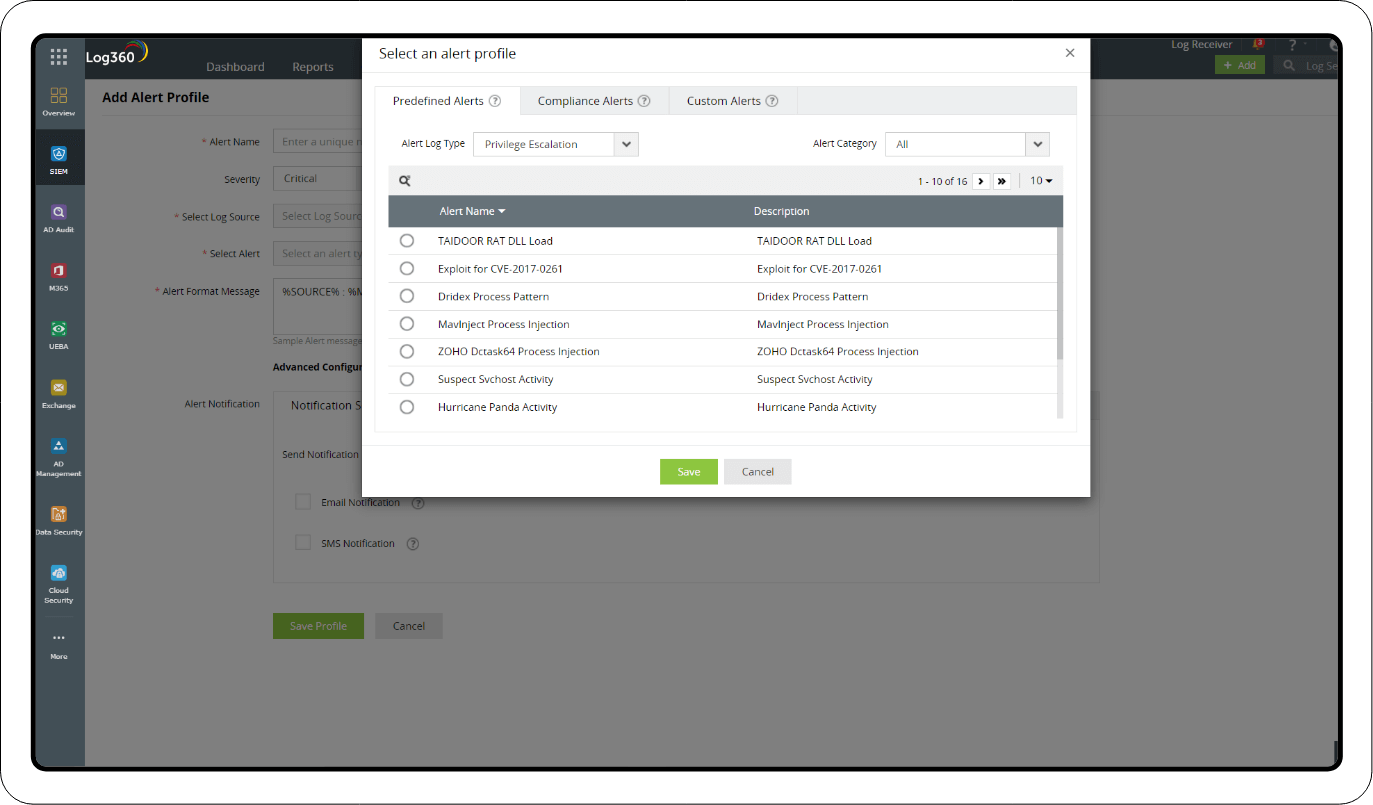The image showcases a laptop screen with a white border. In the top left corner, the Log360 logo is visible, accompanied by various navigation tabs including Dots, Overview, CM, Ad Audit, M365, Ultra, Exchange, Ad Management, Data Security, and Cloud Security. Additional tabs such as Log316, Show Red, Blue, Yellow, Dashboard, and Reports are also present.

Central to the interface, text fields and dropdown menus provide options for setting up an alert profile. These include fields and selectors for "Alert Name," "Enter Unique," "Severity" (with a critical level), "Select Log Source," "Select Alert," "Alert Format Message," "Events Config," and "Alert Notification." Notification options include "Send Notification," with an "Email Notification" checkbox, and a "Smart Notification" feature.

At the bottom of the screen, a green rectangle labeled "Save Profile" and a gray rectangle labeled "Cancel" are present. Further sections allow the user to select alert profiles categorized under "Predefined Alerts," "Compliance Alerts," and "Custom Alerts." Additional categories include "Alert Log Type," "Privilege Escalation," and "Alert Category."

Listed within these sections are various alert examples such as "Teletraan," "DLL," "Low," "Dexploit," "4CB," "JDS Process Pattern," and "JDS Process Injection." The interface also includes "Save" and "Cancel" options for finalizing actions.